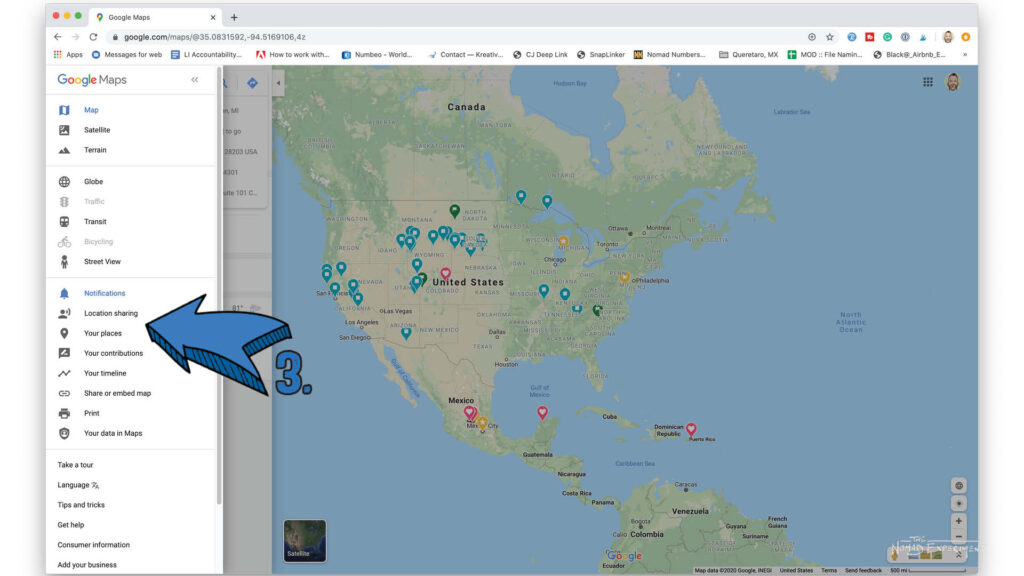The image depicts a web browser window displaying the Google Maps interface. The browser has a gray border at the top, with three distinctive circles on the left: red, yellow, and green. The browser tab reads "Google Maps," and the address bar is visible immediately below along with several icons and bookmarks.

In the main content area, the map showcases the geographical regions of North America, Central America, and parts of South America. Various pushpins are placed on the map, with blue pushpins predominantly located in the United States and red ones scattered across the Caribbean and southern Mexico.

Additionally, a blue arrow annotated with the number "3" and a dot is pointing towards the location sharing section of the Google Maps toolbar on the left side of the screen. This arrow is positioned between the "Your Places" and "Notification" tabs, indicating its importance or relevance to the user.